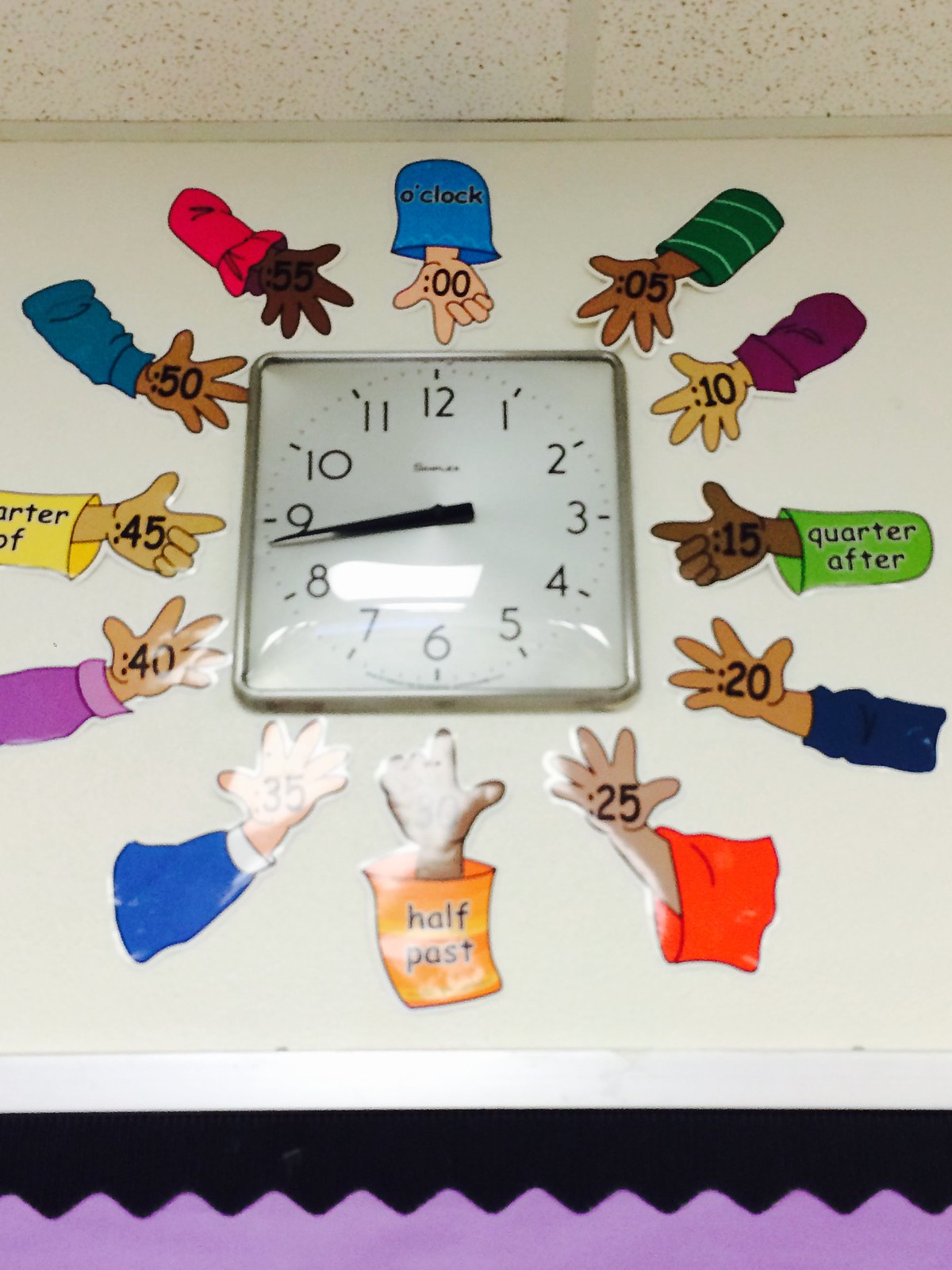This image features a wall clock, likely situated in a school or elementary setting designed to assist in teaching how to tell time. The clock itself is square with a chrome rim, showcasing a classic design with black numerals against a white face and black hands. Surrounding the clock are additional, color-coded hands pointing to specific times, providing detailed annotations for learners. These auxiliary hands include labels such as "zero" at the 12 o'clock position, "5" at 1 o'clock, "quarter after" at 3 o'clock, and "half past" at 6 o'clock. The arrangement serves as a comprehensive, educational display intended to enhance students' understanding of how to read a clock accurately.